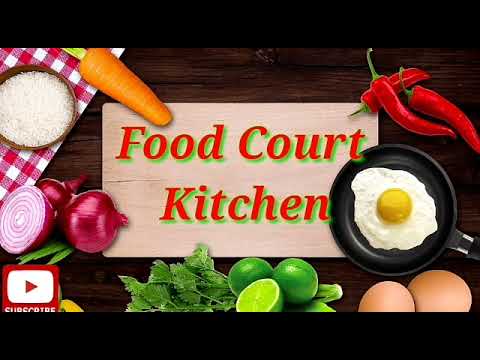The image is a meticulously designed thumbnail for a web show or YouTube channel named "Food Court Kitchen." At the center of the image, there's a light tan rectangle resembling a cutting board, featuring the show's title "Food Court Kitchen" in bold red text with a green glow, set against a backdrop of various food items. The whole composition appears to be a photorealistic mock-up, with food items apparently photoshopped together from different sources.

The food items are arranged on a wooden surface, viewed from a top-down perspective. Starting from the top left, there's a carrot with its green top almost touching the first "O" in "Food." Nearby, there's a bowl filled with rice and a cut-open red onion showcasing its rings. Green beans are placed below the onion, and a small piece of baby corn lies to the right of the YouTube symbol in the bottom left corner.

In the center right, there's a halved lime with two whole limes behind it, flanked by fresh cilantro leaves. Two uncracked brown eggs are situated on the bottom right, adjacent to a small frying pan containing a sunny-side-up egg. Above this, in the top right corner, three red chili peppers are arranged.

The entire image is framed by black header and footer bars, creating a clean and polished look. The YouTube symbol in the bottom left corner, accompanied by the partially cut-off text "Subscribe," emphasizes the promotional intent of the thumbnail, inviting viewers to subscribe to the channel. The image dimensions are approximately five inches wide by four inches tall.